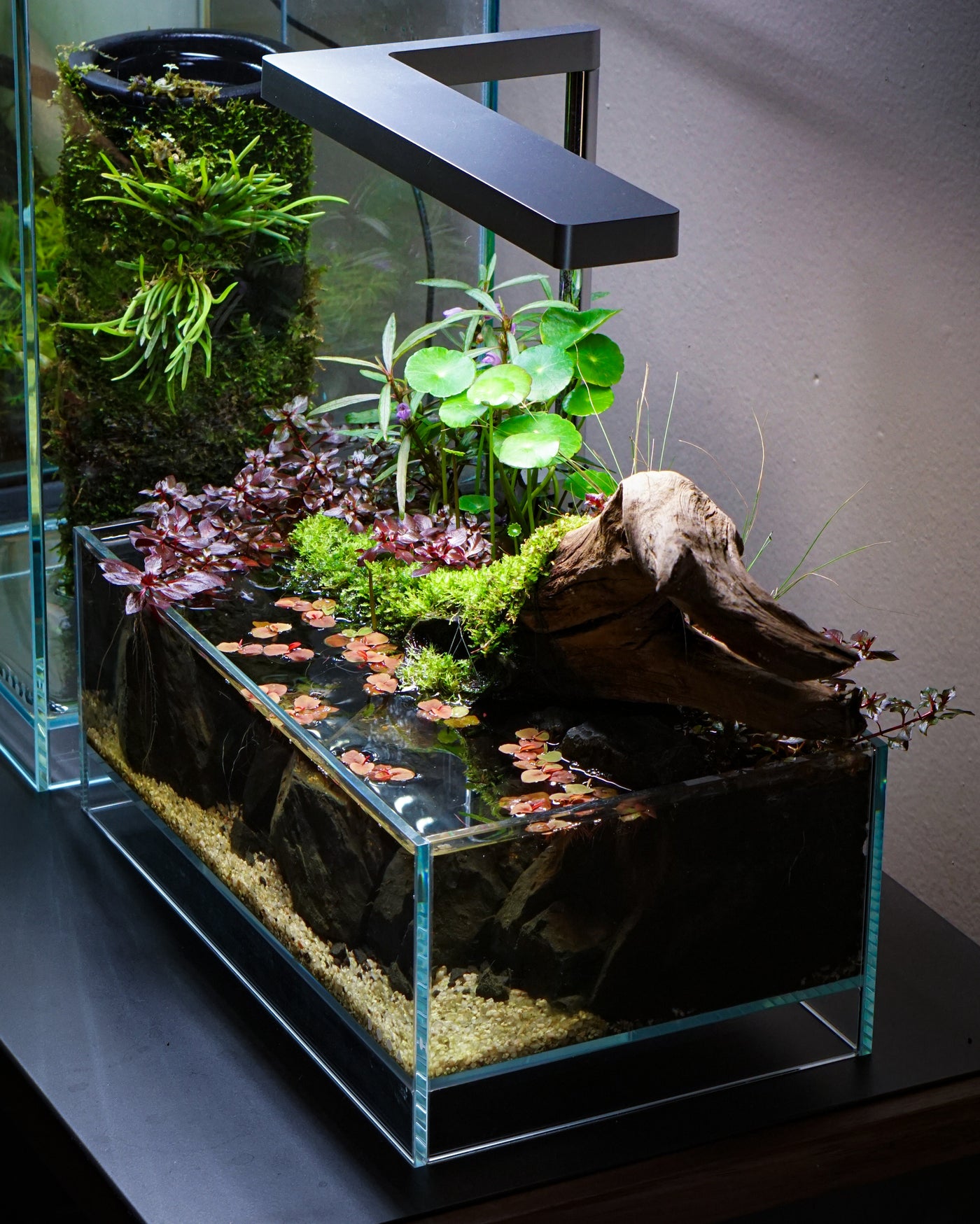This photograph captures an intricate and vibrant terrarium, prominently displayed on a black table. The terrarium itself is a meticulously crafted plexiglass rectangular prism filled with water, with its base layered in a mix of black rocks, brown and tan sand or pebbles, and small white stones. Perched at the top of the terrarium are small, pinkish water lily pads, floating delicately on the water's surface. The scene within the terrarium is further accentuated by the presence of a distinctive piece of driftwood, an ashy-brown addition that adds an organic touch.

A stunning array of plants rises both from within and extends beyond the confines of the terrarium. There are oval-shaped green leaves mingling with vibrant purple plants and patches of light green moss. Some green algae can also be seen within, contributing to the lush, aquatic environment. From certain angles, one can observe branches and sticks submerged in water, contributing to the naturalistic vibe of this water garden. 

A powerful light, reminiscent of a blacklight, illuminates the terrarium from above, casting a surreal glow over the diverse flora. In the background, there's another glass container that appears to hold a vase, from which additional leaves or a viney plant emerge, adding layers of depth to the overall display. The ensemble creates a striking image of a flourishing water garden, teeming with life and color, devoid of any visible fish or animals.